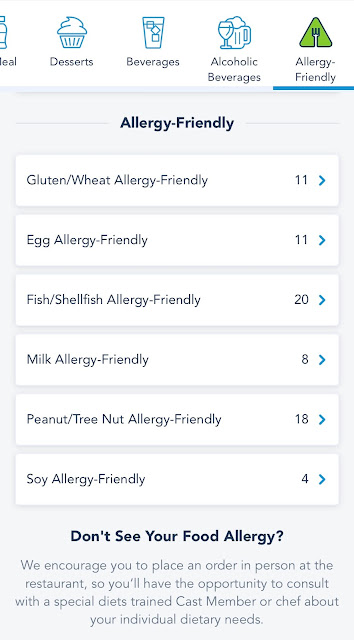Screenshot of a mobile website showcasing dietary options with a focus on allergy-friendly choices. At the top of the screen, there are various icons and corresponding labels serving as headers, displayed in a user-friendly manner:

- A blue cupcake icon labeled "Desserts"
- An icon of a glass with ice cubes labeled "Beverages"
- An icon of a beer mug and wine glass labeled "Alcoholic Beverages"
- An icon resembling a triangle with a fork labeled "Allergy-Friendly"

The website is currently focused on the "Allergy-Friendly" menu, which presents six rectangular cards, each with an arrow on the right for more information. The sections listed are:

1. Gluten/Wheat Allergy-Friendly
2. Egg Allergy-Friendly
3. Fish/Shellfish Allergy-Friendly
4. Milk Allergy-Friendly
5. Peanut/Tree Nut Allergy-Friendly
6. Soy Allergy-Friendly

Beneath these options, a bold black text reads, "Don't see your food allergy?" Followed by gray informational text: "We encourage you to place an order in person at the restaurant so that you'll have the opportunity to consult with a special diets trained cast member or chef about your individual dietary needs."